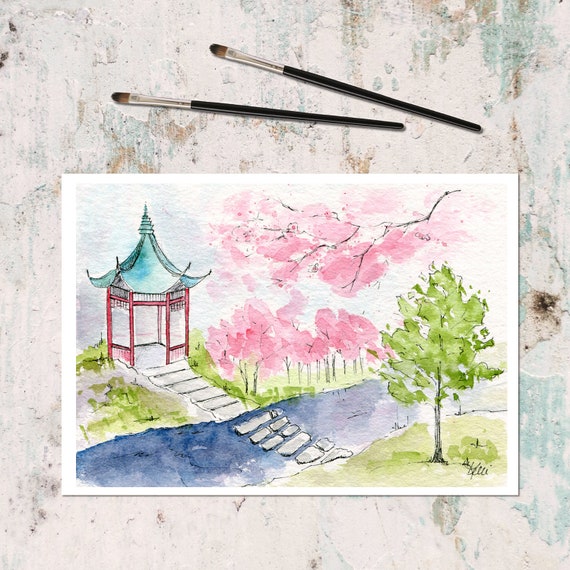The image captures a photograph of a detailed watercolor painting resting on a marble tabletop. The painting showcases a serene scene with a white background and white border. Central to the composition is a pagoda, adorned with a red structure and an aqua blue roof, positioned on the left side of the painting. Surrounding this pagoda are delicate cherry blossom trees, their pink blossoms vividly contrasting against the tranquil setting. 

A picturesque blue river flows through the scene, starting from the left and winding towards the bottom middle right of the image. A stone path, made of white rocks, bridges the river, inviting viewers to imagine crossing over to the pagoda. Nestled on the right bank of the river is a stately tree with a slender gray trunk and flourishing green leaves. 

Above the painting, two paintbrushes with black handles and silver ferrules rest, suggesting the artwork's handcrafted nature. Although the artist’s signature is present, it is illegible. The palette of colors—ranging from the vibrant pink of the blossoms, the serene blue of the river, to the lush green of the grass—creates a harmonious and eye-catching contrast, adding to the painting’s charm and beauty.